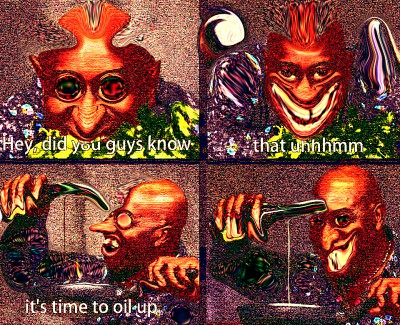The image is divided into four well-spaced quadrants arranged in a windowpane style format, reminiscent of a comic strip, and appears to be a satirical meme commonly seen on social media. The character featured in all four quadrants is an animated, bald creature with distinct red skin, pointy ears, bifurcated hair, a large red nose, and big red eyes. He is dressed in a yellow outfit accented with purple. The image has an intentionally grainy texture. 

In the upper left quadrant, the character is shown from the front with a maniacal smile, saying in white letters, "Hey, did you guys know." In the upper right quadrant, he appears again, smiling widely with a hint of malevolence, with text beneath him spelling out, "UHHMM." 

In the lower left quadrant, the character is depicted in profile, holding something, with his mouth open, revealing snaggle-teeth and a partially missing head. The text states, "It's time to oil up." Finally, in the lower right quadrant, the character is seen pouring oil into a pan, holding the bottle with one hand and the pan with the other, while displaying a devious smile with big white teeth. The colors prominently featured in the image include red, orange, yellow, black, white, gray, and various shades of green.